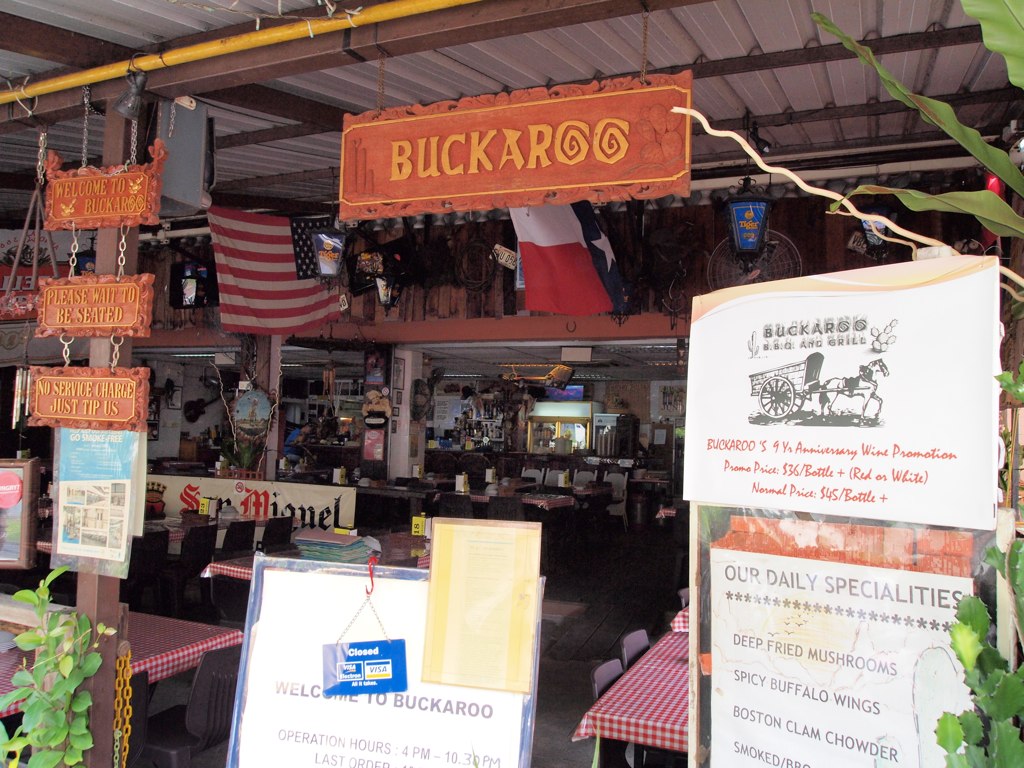The image is of an indoor scene at a restaurant called Buckaroo, which has a lively and colorful décor. Dominating the top center of the image is a large, orange sign with yellow letters spelling "Buckaroo," where the O’s are playful swirls. To the left of this sign, three smaller signs hang from chains, reading "Welcome to Buckaroo," "Please wait to be seated," and "No service charge, just tip us." Beneath these signs, both an American flag and a Texas flag are suspended from the ceiling, adding to the thematic ambiance.

In the center of the image, a menu board prominently displays a blue "Closed" sign, with a larger white sign beneath it saying "Welcome to Buckaroo" and listing operation hours from 4 p.m. to 10:30 p.m. On the right side of the image, a poster for Buckaroo's Barbecue Grill announces their fourth anniversary wine promotion and lists daily specials such as deep-fried mushrooms, spicy buffalo wings, Boston clam chowder, and smoked barbecue.

Scattered throughout the room are tables covered with red and white checkered tablecloths, each equipped with napkin holders. An additional half-visible sign to the back reads "San Miguel." The overall atmosphere, filled with vibrant signage and eclectic décor, suggests a venue that’s both a restaurant and possibly a roadside attraction or souvenir shop, designed for fun and welcoming gatherings.